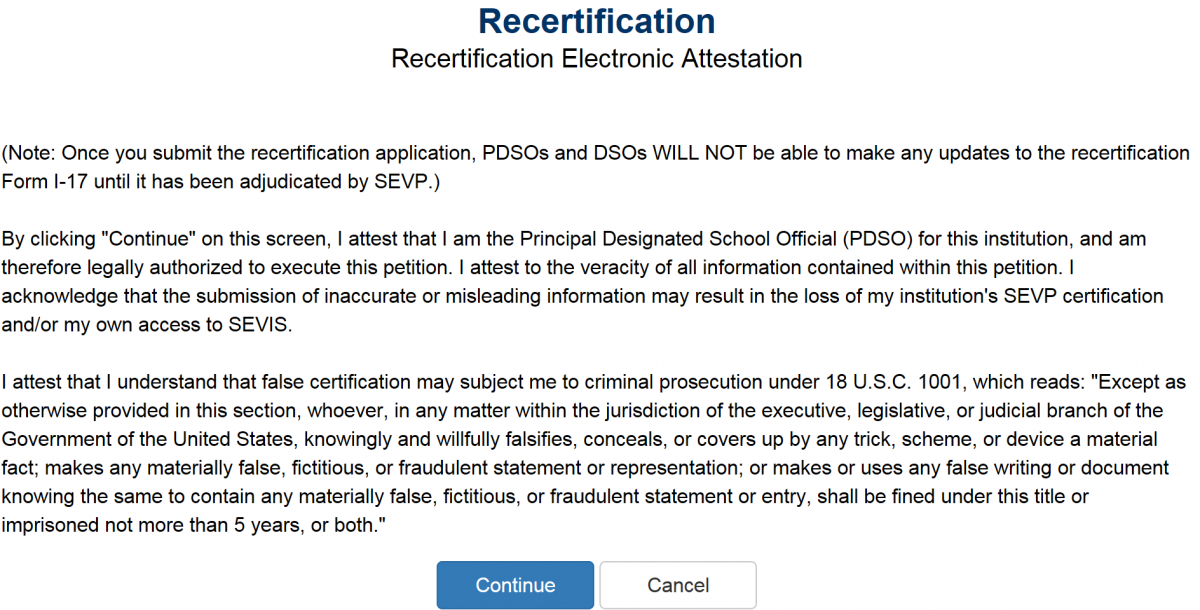**Recertification Electronic Attestation Form**

---

*Top Center Text - Bold and Large Font: "Recertification"*

*Subheading - Bold, Smaller Font: "Recertification Electronic Attestation"*

The form consists of three main paragraphs with detailed instructions and legal affirmations, followed by two buttons at the bottom: a blue "Continue" button and a white "Cancel" button.

**Paragraph 1** *(entirely in parentheses)*:
*(Note: Once you submit the recertification application, Principal Designated School Officials (PDSOs) and Designated School Officials (DSOs) will not be able to make any updates to Recertification Form I-17 until it has been adjudicated by the Student and Exchange Visitor Program (SEVP).)*

**Paragraph 2**:
By clicking on the "Continue" button, you attest that:
- I am the Principal Designated School Official (PDSO) for this institution.
- I am legally authorized to execute this petition.
- I attest to the veracity and accuracy of the information contained in this petition.
- I acknowledge that the submission of inaccurate or misleading information may result in the loss of the institution's SEVP certification and/or my access to the Student and Exchange Visitor Information System (SEVIS).

**Paragraph 3**:
I understand and attest that providing false certification may subject me to criminal prosecution under 18 U.S.C. 1001, which states:
- *(Except as otherwise provided in this section, whoever, in any matter within the jurisdiction of the executive, legislative, or judicial branch of the Government of the United States, knowingly and willfully falsifies, conceals, or covers up by any trick, scheme, or device a material fact, makes any materially false, fictitious, or fraudulent statement or representation, or makes or uses any false writing or document knowing the same to contain any materially false, fictitious, or fraudulent statement or entry, shall be fined under this title or imprisoned not more than five years, or both.)*

**Buttons at the Bottom**:
- *Blue "Continue" Button*
- *White "Cancel" Button*